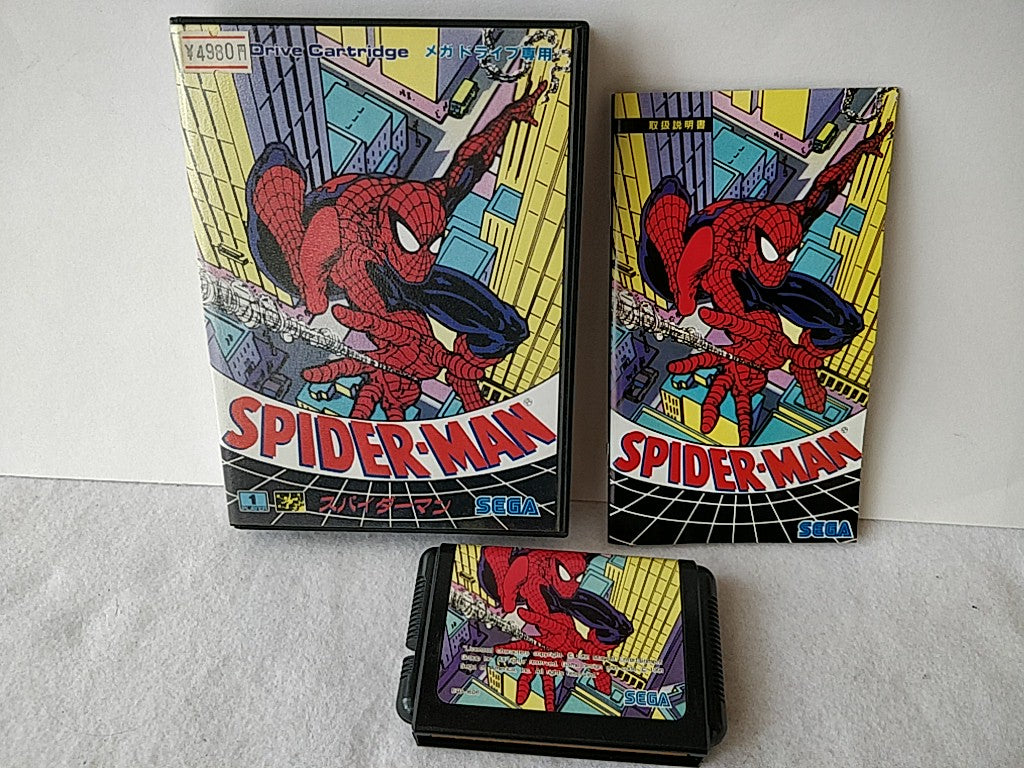In the picture, there's a gray carpet on the floor, noticeably wrinkled in certain spots, indicating wear. Placed centrally on this carpet is a black container adorned with a vibrant Spider-Man image. This image depicts Spider-Man perched atop city skyscrapers, spinning a web from one hand behind him, while the other hand is stretched forward. The background features a mix of yellow and blue buildings. The container prominently displays the Sega logo at its base.

Adjacent to this scene, two larger Spider-Man themed CD-like boxes lean against a light gray or opal-colored wall. These boxes showcase the same Spider-Man artwork, with additional details. One box includes a label with the number "4980" and the phrase "drive cartridge" along with text in Chinese or Japanese, all set within a black box with yellow text. The other box similarly features Asian text in blue on the left side. Both boxes also carry the Sega branding, linking them to the black container on the floor.

This detailed depiction suggests that these items might be video games or related merchandise, designed for children, combining vibrant imagery with recognizable branding and multilingual text.